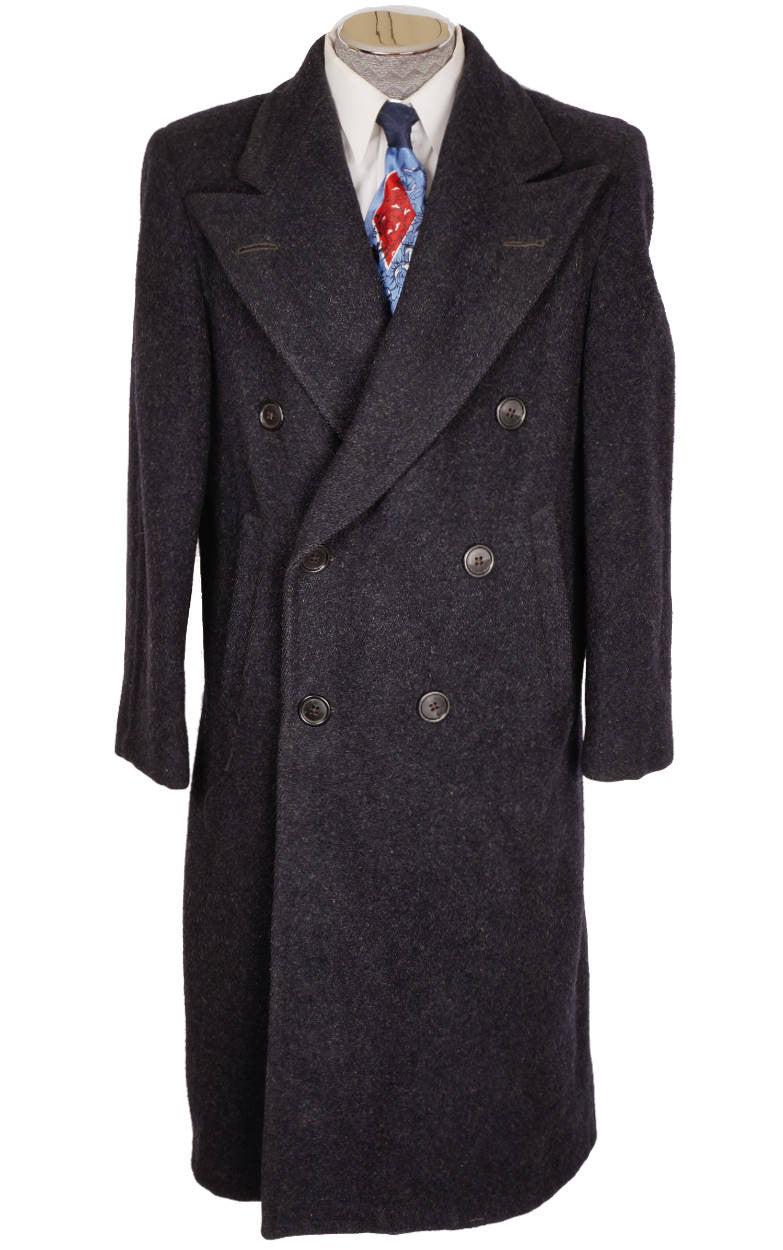This photo showcases a low-resolution image of a black, wool long coat that extends from the neck to knee height. The coat, which appears to be hanging on a headless mannequin, features a double-breasted design with six buttons on the left front side and three buttons on the right. Underneath, a collared white dress shirt is visible, paired with a dark blue tie adorned with a light blue and red diamond pattern. The overall ensemble suggests it may be a second-hand item potentially being sold online, and the coat itself has long sleeves made of a felt-like fabric. The background of the image is transparent, further emphasizing the focus on the clothing.